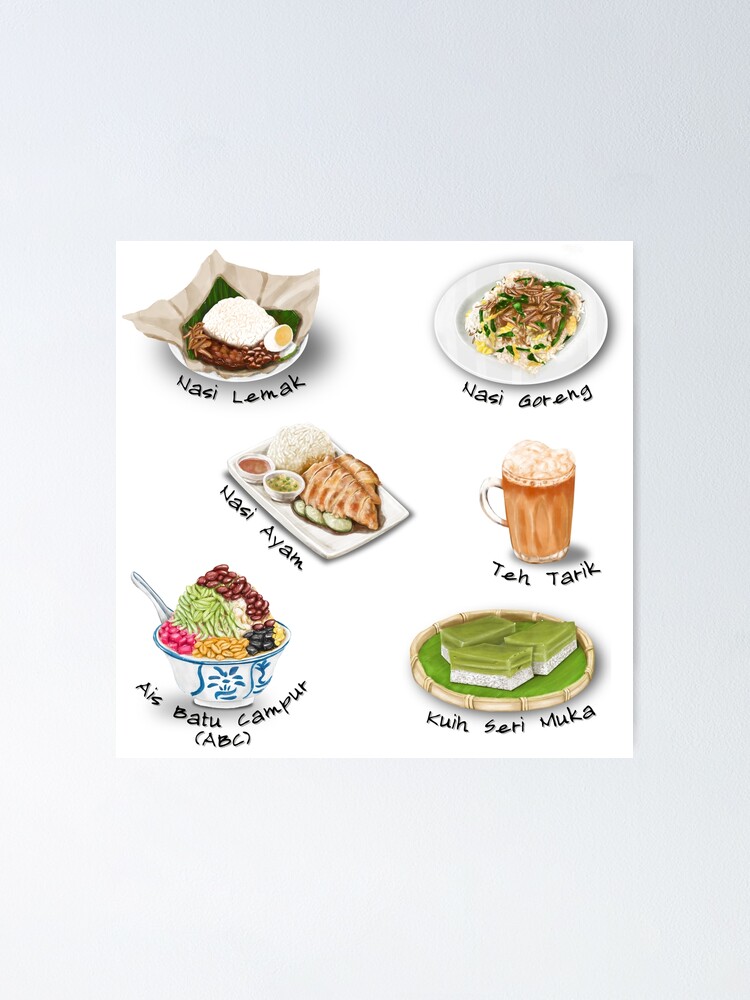The advertisement, which appears to be a hand-drawn menu on a white background with Asian stylistic elements, showcases six items available at the restaurant. 

1. **Nasi Lemak**: This dish includes a bowl of rice, a boiled egg cut in half, and green vegetables, possibly seaweed or lettuce.
2. **Nasi Goreng**: A fried rice dish adorned with onions, mushrooms, and bean sprouts.
3. **Nasi Ayam**: Comprising rice, chicken, and various condiments or dips.
4. **Teh Tarik**: A traditional tea drink, resembling a mug of root beer with a white foam on top.
5. **Ais Batu Kampur (ABC)**: A dessert with various types of beans, nuts, and presumably rice.
6. **Kuih Seri Muka**: A green and white layered dessert.

This colorful and detailed poster effectively advertises the diverse selection of Asian dishes and drinks offered by the restaurant.